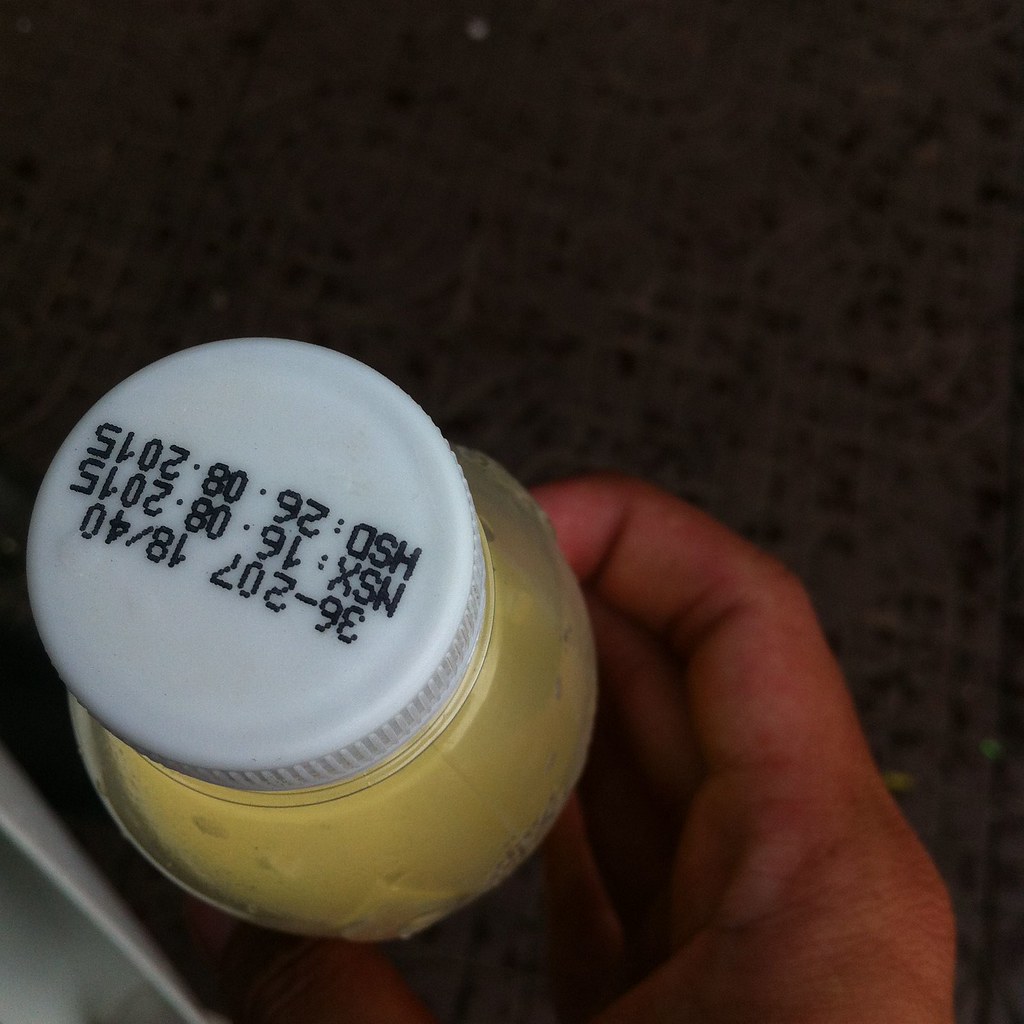This image captures a detailed close-up of a clear plastic bottle with a white, indented screw cap, held by a right hand in the bottom right corner. The bottle, containing a yellow liquid, is stamped with various numbers and letters, including "36-207-18-40 NSX-1608-2015, HSD-2608-2015." The background is a black, possibly carpeted fabric with visible textures and small holes, potentially resembling burlap. In the lower left corner, a portion of a curved white object is visible against the fabric.